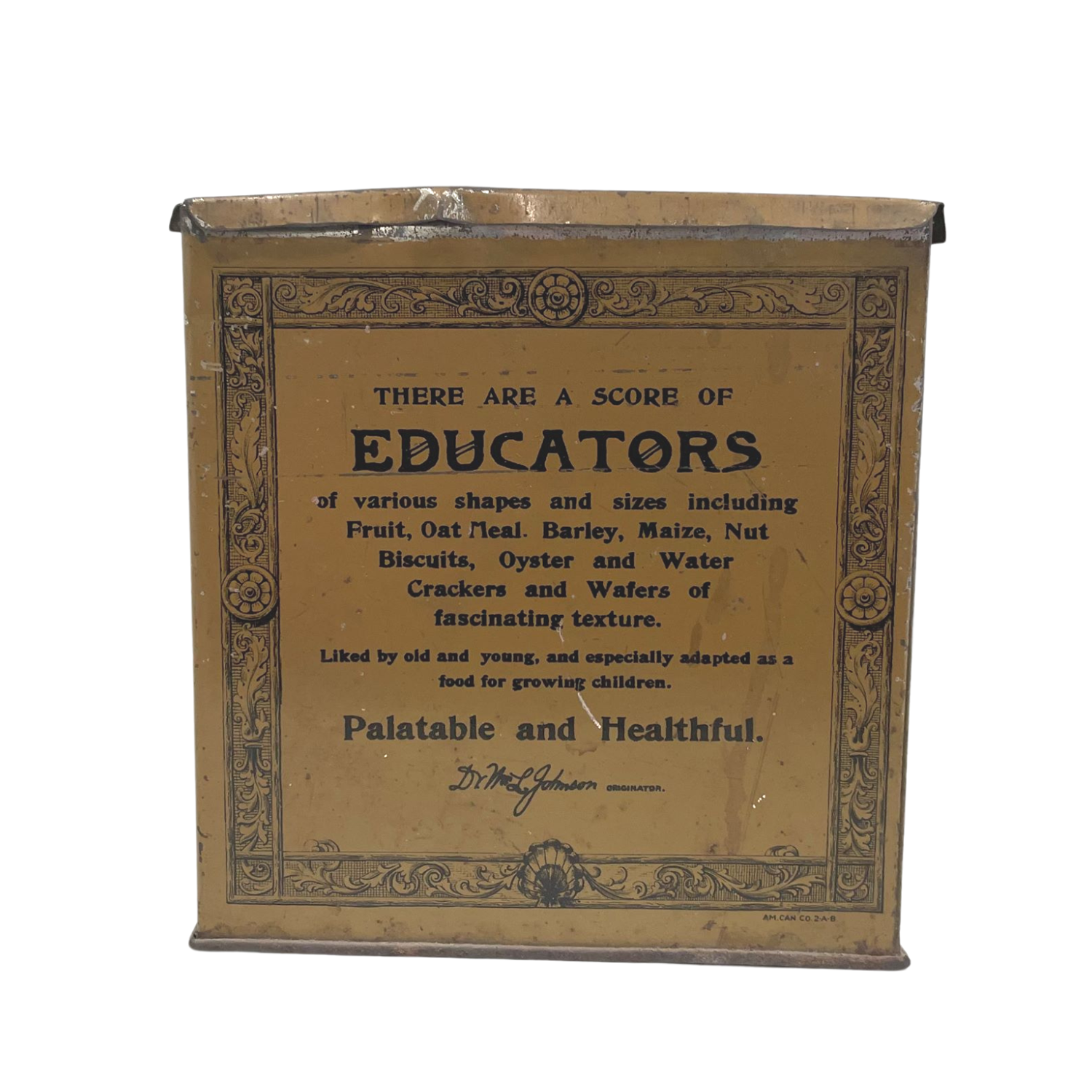The image depicts a weathered, metal plaque or tin with a corroded brown appearance, showcasing clear signs of age such as water stains, scratches, and chipped paint. The item has a somewhat official 19th-century look, enhanced by a plant-themed decorative border encasing the central text. This text proclaims: "There are a score of educators of various shapes and sizes, including fruit, oatmeal, barley, maize, nut, biscuits, oyster, and water crackers and wafers of fascinating texture, liked by old and young, and especially adapted as a food for growing children, palatable and healthful." Beneath this text, there is an unreadable cursive signature followed by the word "originator." The top of the plaque or tin appears bent, adding to its vintage and rugged character.